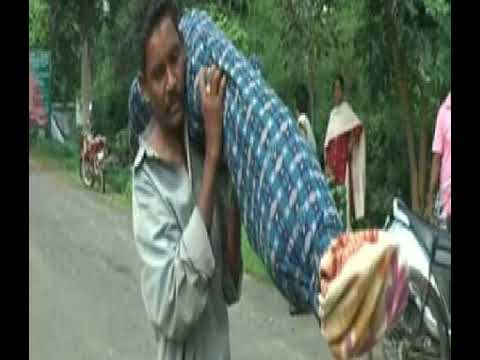The image appears to be a low-resolution, slightly blurry screen capture of an outdoor scene, possibly taken from a TV or monitor, with black borders on the left and right sides. In the center of the image, a dark-skinned man with black hair walks along a concrete path. He is wearing an oversized, unbuttoned, long-sleeved gray shirt with cuffs and holding what appears to be a blue rug draped over his left shoulder. The rug features a blue, light blue, and white plaid pattern, and there seems to be some colorful fabric, possibly yellow, orange, and purple, visible at one end, potentially suggesting it could be wrapped around something significant.

In the background, there is a tree-lined area with green grass and several people standing around. Notable among these individuals are a woman in a red floral dress with a white scarf and a man in a white shirt with his back turned. To the right of the central figure is a parked bicycle, and further to the right, motorcycles are also visible. The scene suggests a gathering of some kind, possibly a somber event, given the way the rug is being carried.